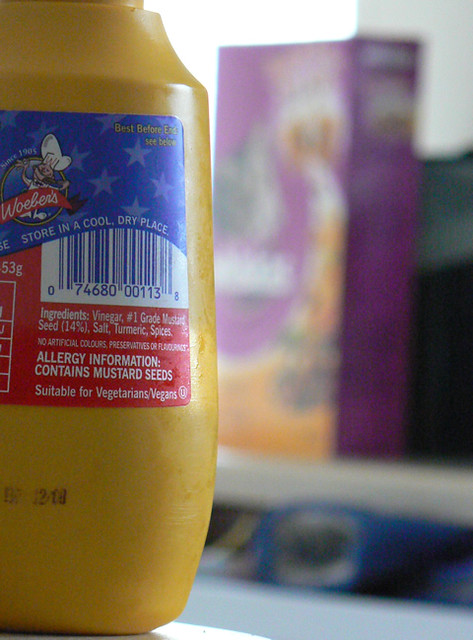This is a close-up image of a yellow plastic mustard bottle, prominently featuring the brand name, which seems to be Willoughby's or Wobbles, though it's not entirely clear. The focus is on the left-hand side of the bottle, highlighting its intricate label. The label is adorned with a cartoon chef in an elaborate hat that appears to be dancing, set against a blue background with American-style stars. Above the white UPC tag with blue vertical stripes, it reads "Store in a cool, dry place" and "Best before" followed by a date. The red section of the label includes detailed ingredients such as vinegar, number one grade mustard seed, salt, turmeric, and spices. It also provides allergy information, stating it contains mustard seeds, and notes that it is suitable for vegetarians and vegans. Behind the sharply focused mustard bottle, the image blurs, revealing indistinct objects including a potentially purple boxed item, perhaps cereal or another packaged food item.